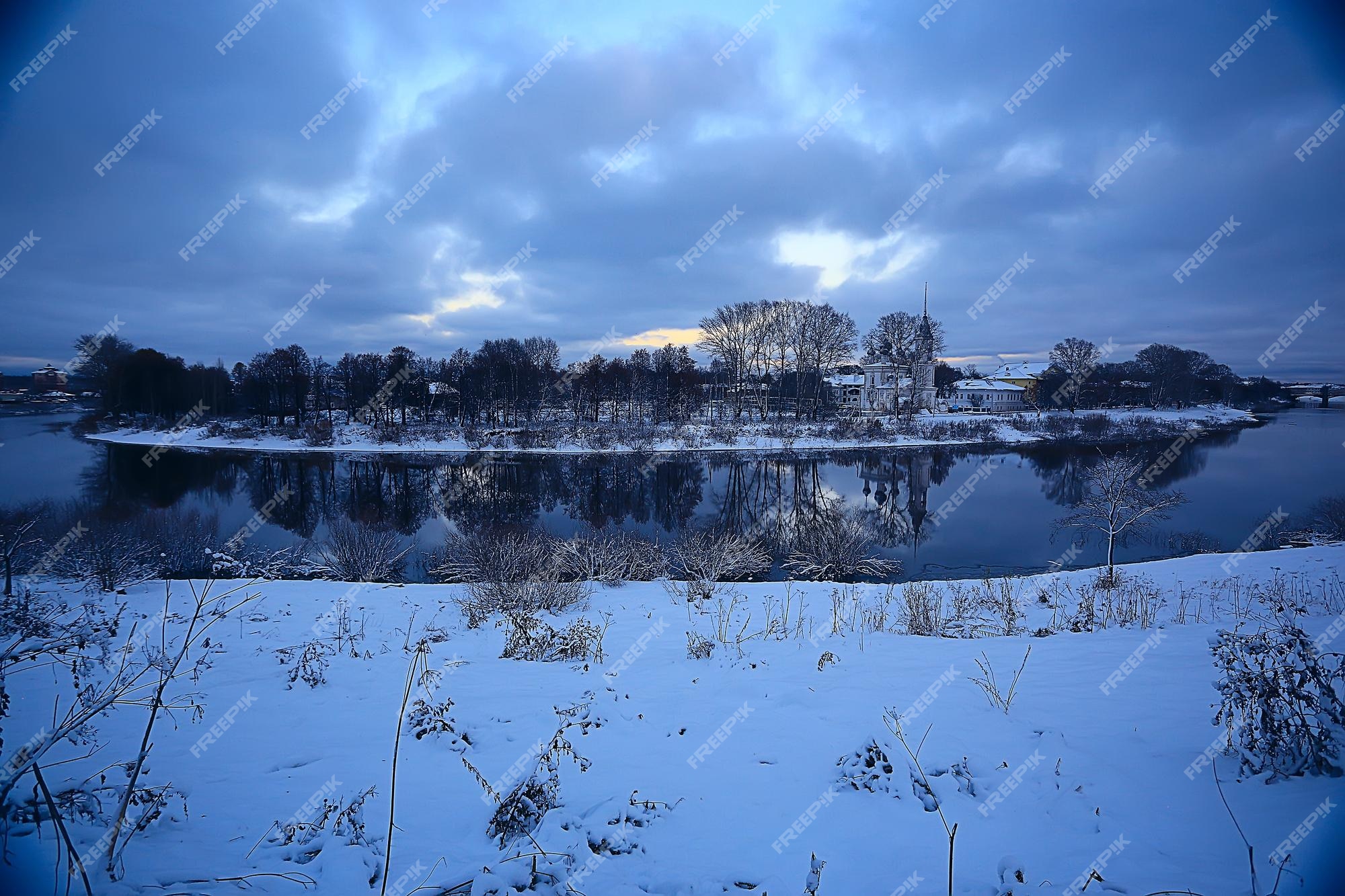The photograph captures a tranquil winter scene by a lake that appears to be in the later stages of dusk or early morning. The sky is heavily clouded, with patches of sunlight piercing through, casting a soft glow over the landscape. The water of the lake is a clear, reflective surface that mirrors its surroundings. A bed of snow covers the foreground, scattered with small patches of dead foliage, none larger than a small chihuahua. In the middle of the lake rests an island adorned with tall, bare trees and blanketed in snow. In the distance, behind these trees, several snow-covered houses are faintly visible. Adding to the picturesque quality, a steeple—possibly belonging to a church—protrudes from the background. The scene exudes a serene, wintry calmness as the day transitions into night, accentuated by the icy stillness of an outdoor setting in the cold.